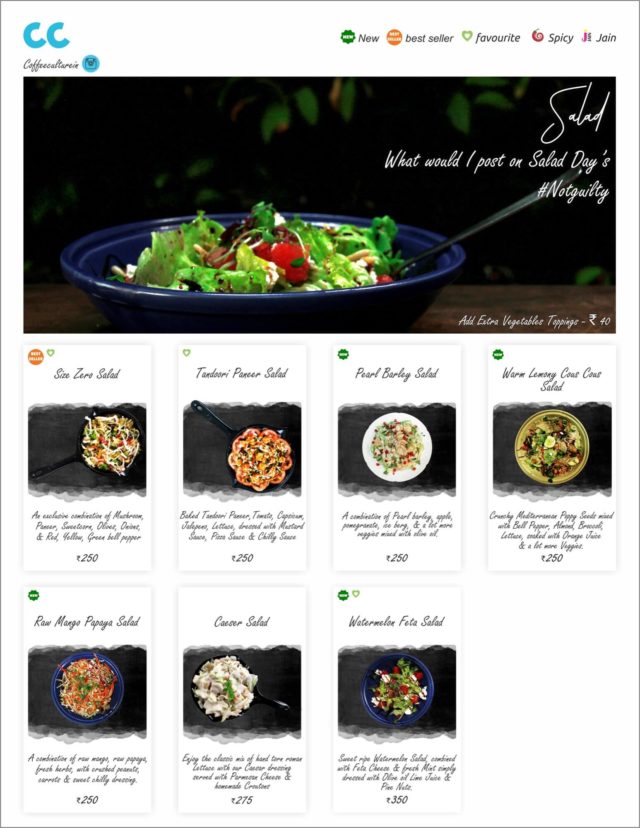This is a screenshot of a website created by CC, showcasing a selection of gourmet salads. The featured image on the site highlights a vibrant, fresh salad served in a blue bowl with a fork neatly resting on the side. The salad is a medley of crisp greens and ripe red tomatoes, all lightly tossed in a speckled dressing, making it visually appetizing. 

At the top of the website, bold text categories such as "New," "Best Seller," "Favorite," and "Spicy" are prominently displayed, alongside an option for visitors to join the community. Below these categories, the website extensively features an array of seven distinct salads, each beautifully photographed against a sleek black background. The salads vary in composition, with some emphasizing rich greens while others highlight vibrant reds. One particularly eye-catching dish is a pristine white Caesar salad. Another unique offer is a creatively named 'Watermelon Feta Salad.'

The website appears to specialize in salads, though further investigation of the menu would be required to determine if other types of cuisine are available. Regardless, the salads are undeniably the stars of the site, with each one meticulously described and visually presented to entice potential diners.